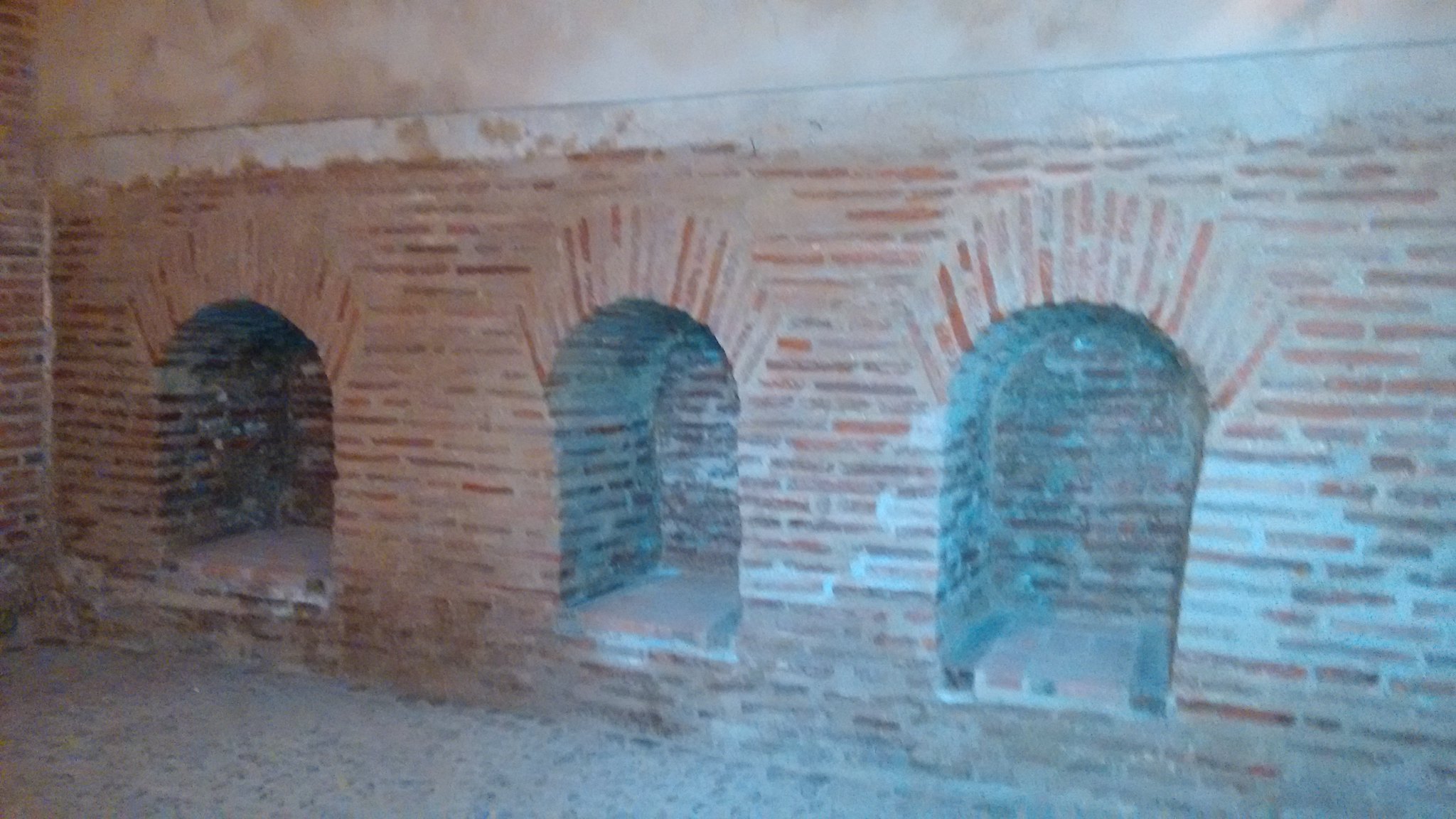The photograph, slightly out of focus and possibly old, depicts a horizontally rectangular frame of what appears to be a basement or indoor setting. The main feature is a red brick wall showcasing three arched alcoves. The bricks are varied in shades of red, leaning towards dark reddish brown. Each archway is meticulously constructed with vertically standing bricks, creating a distinctive pattern. The alcoves are not very deep and have small square terracotta tiles at their bases. Above the brick wall, a cement section seamlessly integrates with a narrow border separating it from the brick. The floor, visible at the bottom of the frame, consists of either cobbled stones or small bricks. A similar brick pattern extends to a section of the left wall. The alcoves, devoid of any statues or objects, seem purpose-built for display, adding an intriguing architectural detail to the setting.